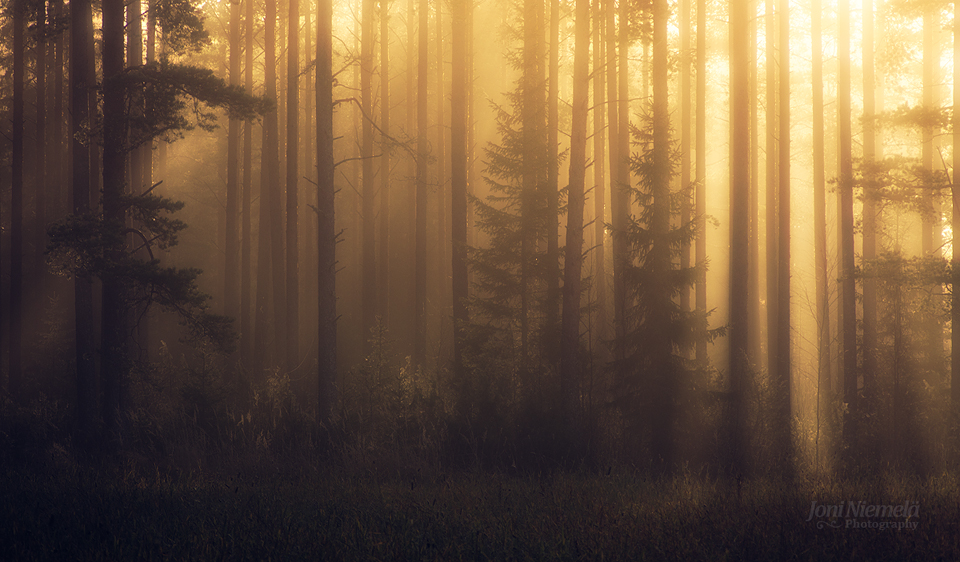This professional photo by Jeanne Niemeld captures a mystical forest scene bathed in an amber hue. Tall, slender pine trees dominate the frame, their dark silhouettes creating a striking contrast against the softly shining sunlight filtering through the dense forest canopy. The sunlight, originating from the top right corner, casts golden rays that gradually blend into darker shades towards the bottom left, where the forest floor becomes nearly indiscernible in deep shadows. Some of the trees are bare, their intricate branches forming almost sketch-like outlines against the background. The scene is both ethereal and haunting, with the forest floor covered in a lush carpet of grass in the foreground. Jeanne Niemeld Photography is subtly inscribed in transparent font at the bottom right corner, adding a professional touch to this enchanting woodland image.